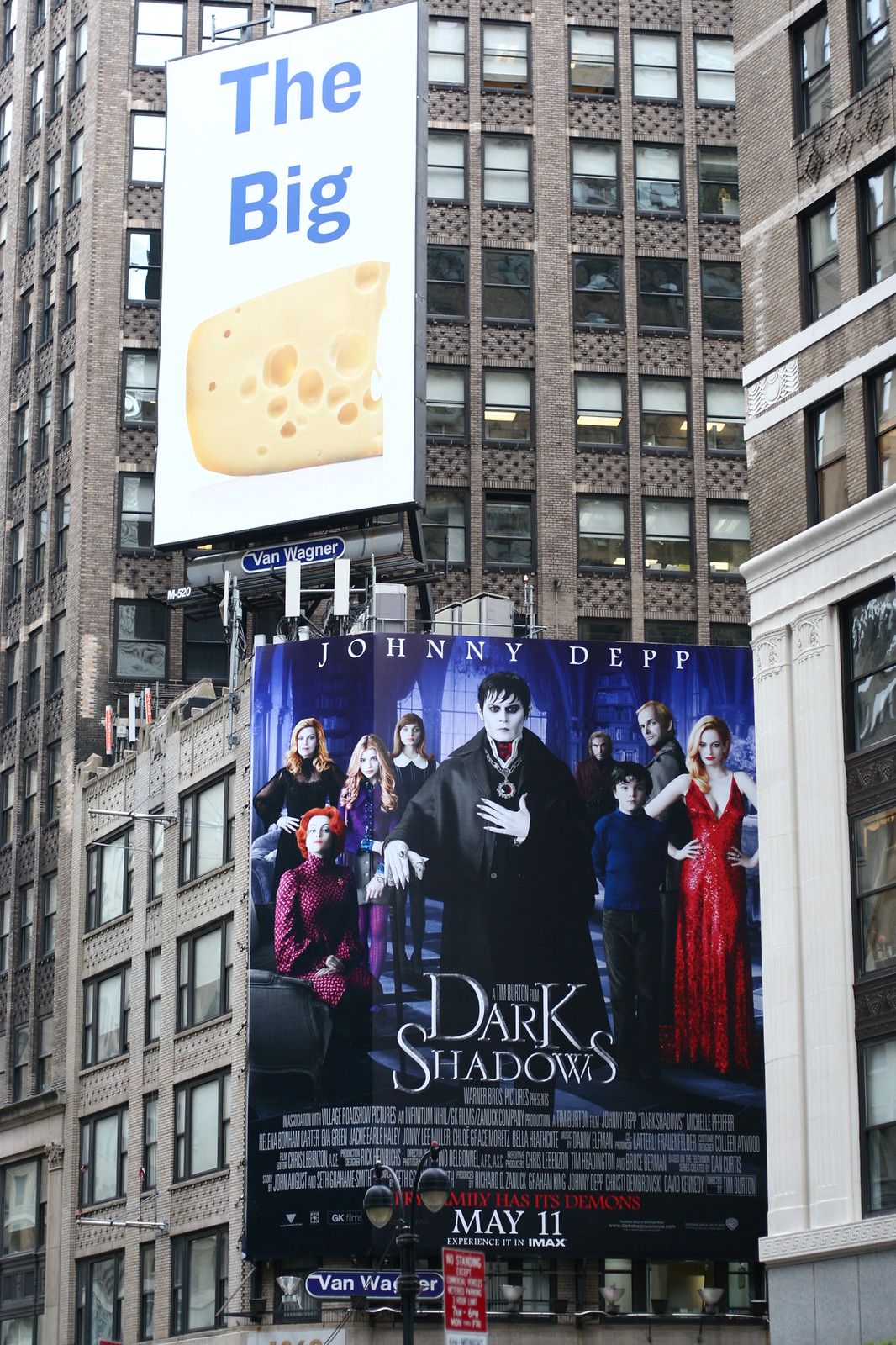The image captures a large tan building adorned with numerous windows. Prominently featured are two signs affixed to the side of the building. In the upper left corner, a rectangular sign with a white background displays large blue lettering that reads "The Big," accompanied by an image of a Swiss cheese wedge below the text.

Beneath this sign is a larger movie poster for the film "Dark Shadows." The poster showcases the cast with Johnny Depp prominently positioned at the center, dressed as a vampire. The background of the poster is blue. Across the top, "Johnny Depp" is written in white, while the movie title "Dark Shadows" is centered in bold white letters. At the bottom of the poster, the release date "May 11th" is also displayed in white.